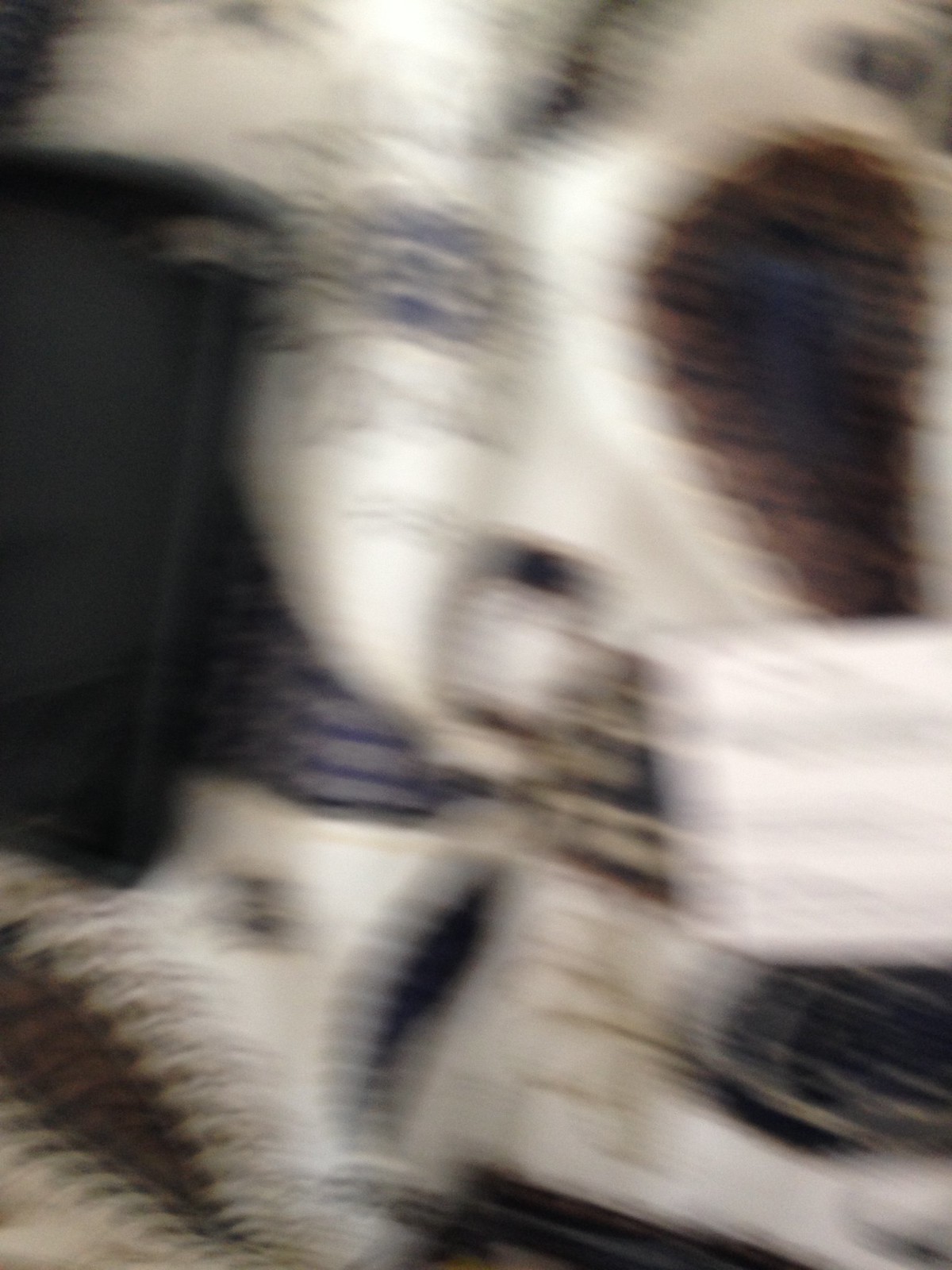The painting is an abstract, slightly blurred composition predominantly in shades of black and white, with some sepia tones. It features large blocks of black and white with varying degrees of shading, creating an unclear and out-of-focus effect. Intriguingly, the more you examine the painting, the more details you begin to notice. Scary, distorted faces emerge from the abstract shapes, including a baby doll-like face with one eye open in shock and a darkened area where the other eye should be, resembling a ghostly visage. Another potential face with one eye is discernible below. Amidst the curvy and rounded shapes, there are sections that give the impression of a fur-like texture, and a zipper-like design appears on the bottom left. A large, sepia-toned oval shape, possibly a head, is visible on the right, while a significant square form occupies the left. The combination of these elements creates a haunting, enigmatic image that continually reveals new, eerie details.